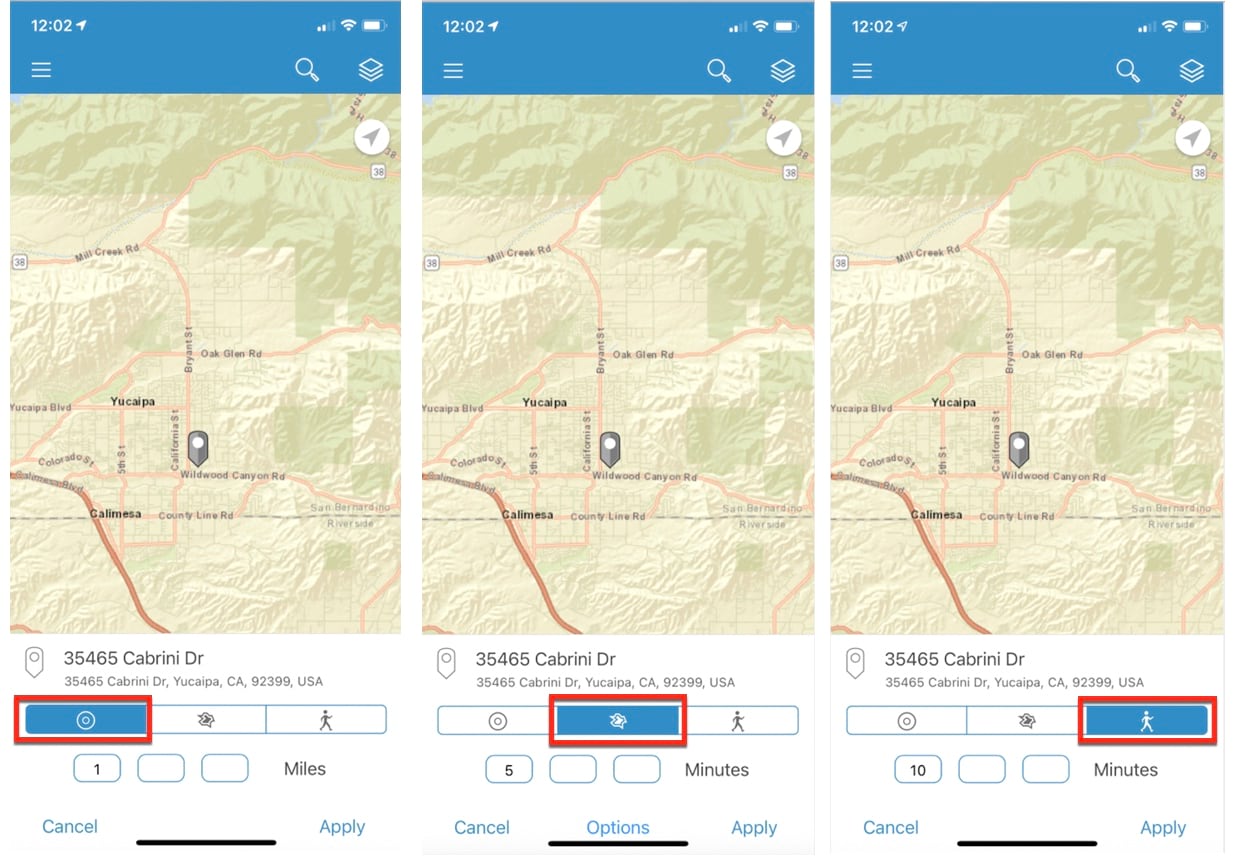The image depicts three side-by-side screenshots of a cell phone, each showcasing identical user interfaces and content. Each screenshot features a blue header at the top, indicating the time of 12:02 in the upper left-hand corner. Adjacent to the time, on the right side, are icons representing signal strength, Wi-Fi availability, and battery power, all showing around 90% charge.

Beneath these indicators, the screenshots display icons for menu options, a search functionality represented by a magnifying glass, and what appears to be an icon for different map layers. The main part of the screenshots is occupied by a detailed elevation terrain map of a town, predominantly colored in light green, yellow, and beige, with red or pink roadways. The map includes labels such as "Yucaipa," possibly indicating the town’s name, and street names like "County Line Road" and "Mill Creek Road."

Below each map, the address "35465 Cabrini Drive" is written in black font, with additional details including "Yucaipa, CA 92399, USA" in gray font. Further down, three icons are displayed, with one shaded in blue and the others in white, depicting a person walking among other illustrations. Additional information about distances in miles is provided below these icons.

At the bottom of each screenshot, there are options to "Cancel" on the left and "Apply" on the right, both in blue font, separated by a black bar in the middle.